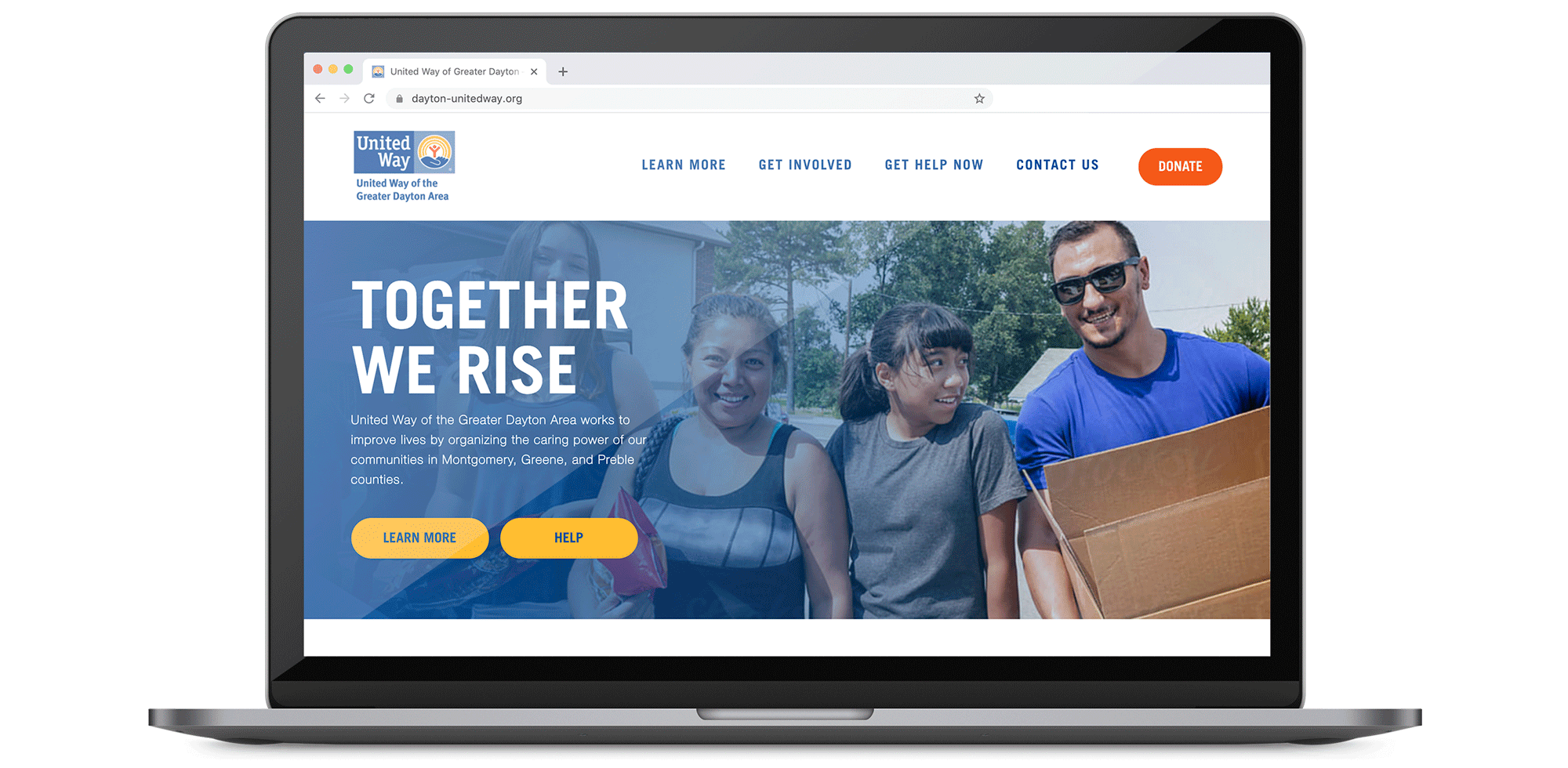This photograph displays a Mac laptop showcasing a website for United Way. The silver laptop has a black bezel around the screen, which prominently features a webpage. The webpage, which looks like it could be part of a slideshow presentation, has a striking photograph that occupies about three-quarters of the page, with a blue filter gradient that is more intense on the left side. 

Across this photograph, large white text declares "Together We Rise." Below this, a four-line paragraph of smaller text provides additional context. Beneath the paragraph, there are two yellow buttons with blue text: the left one reads "Learn More," and the right one says "Help."

The depicted photograph includes four individuals: three women on the left side and a man on the right side, who is wearing sunglasses, a blue t-shirt, and carrying a cardboard moving box. Just above the photo, the United Way logo is visible on the left side of the page.

The site’s menu has a white background with blue text, and includes options such as "Learn More," "Get Involved," "Get Help Now," and "Contact Us." On the right corner, there's an orange box with the word "Donate" prominently displayed.